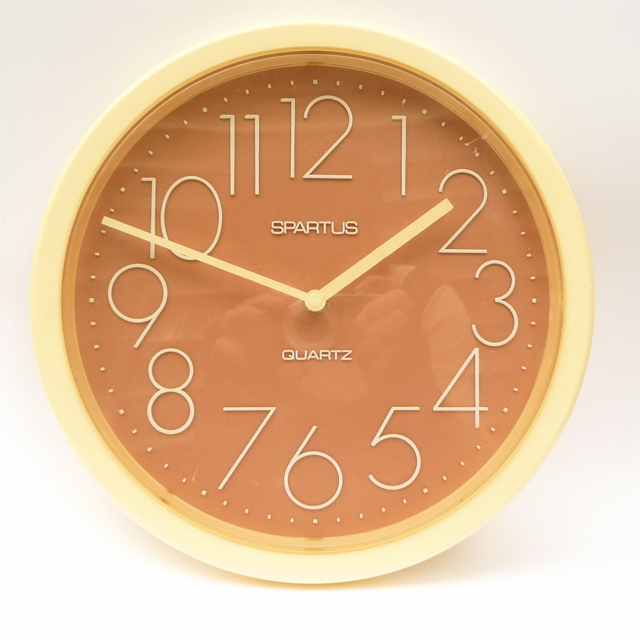This image depicts a Spartus quartz wall clock, prominently featuring the brand name "Spartus" above the central hands and "quartz" below. The face of the clock is a creamy light yellow hue, while the clock face itself sports a pale brown, almost chocolate color. The white-colored numbers and minute marks encircle the dial, with exaggeratedly large digits set against subtle, every-minute white dashes and slightly emphasized five-minute markers. The pale yellow, rectangular hour and minute hands of the clock show a time close to 1:48. A glass cover over the clock creates a reflective surface, capturing the faint image of the photographer. The clock casts a drop shadow, suggesting it may be laying flat rather than hanging on a wall. The background appears to be a plain white wall, highlighting the clock's design and details.